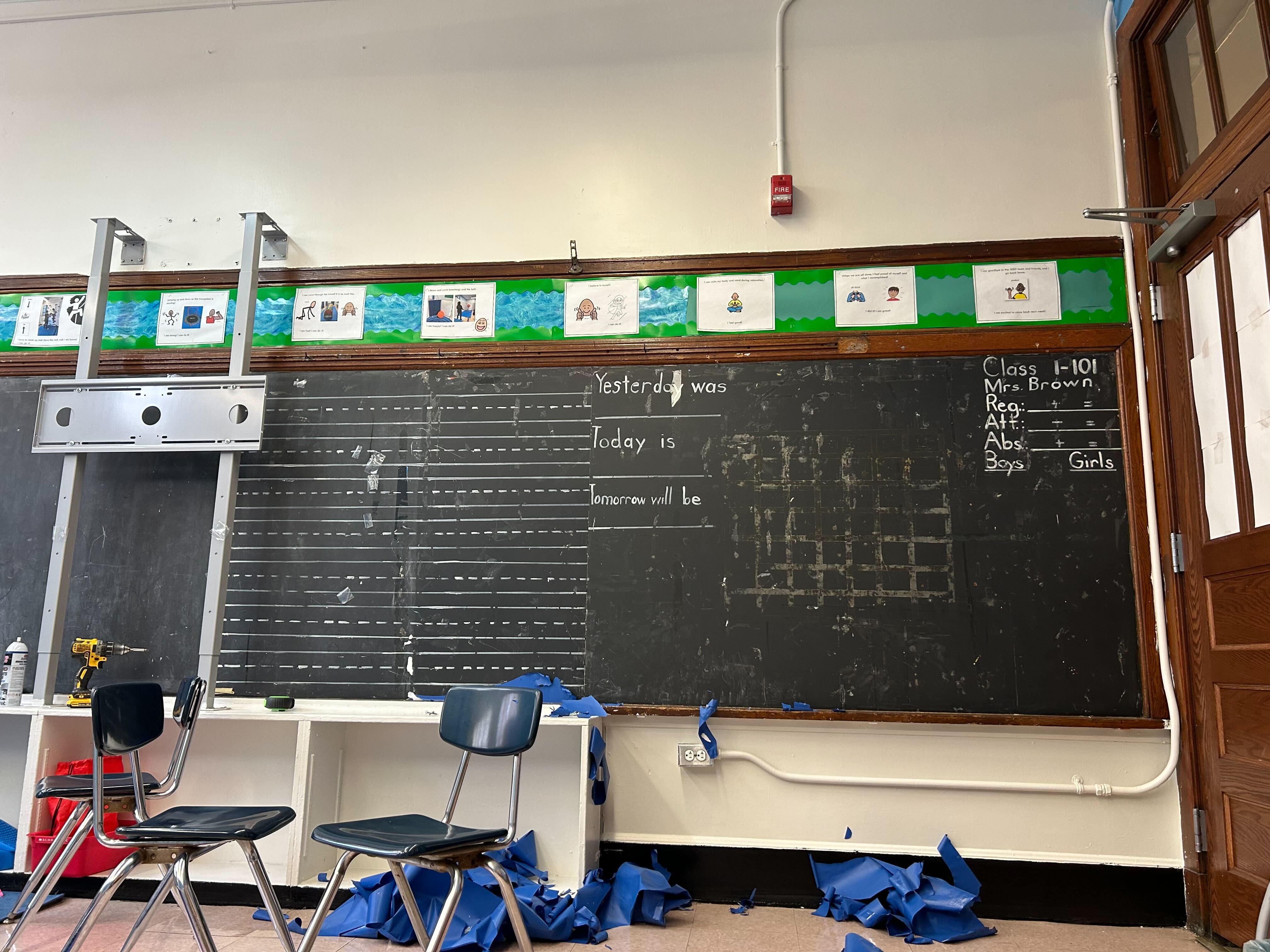This detailed photograph captures a nostalgic glimpse inside an old classroom, focusing on a timeworn chalkboard. The chalkboard is central to the image and bears visible signs of age, with various markings and old tape residue stubbornly clinging to its surface. In the top left corner, written in chalk, are the words: "REG, Yesterday Was Blank, Today Is Blank, Tomorrow Will Be Blank." The top right section of the chalkboard reads: "Class 1-101, Mrs. Brown, REG, ATT, ABS, Boys, Girls," detailing a typical classroom overview.

The center of the blackboard resembles a large sheet of notebook paper, adorned with numerous white lines imitating pages. Below, scattered blue paper remnants lie on the ground, evidently torn from the chalkboard at some point. Adding to the scene of abandonment or transition, a mount intended for a television or projection screen is affixed to the left side, connected to a small white cubby attached to the wall.

In the foreground, the classroom floor is strewn with chairs, particularly gathering towards the left corner, suggesting a state of disarray. A drill and a canister, likely spray paint, rest on one of the tables to the left, implying ongoing renovation or deconstruction efforts. This detailed setting evokes a sense of change, reflecting either a remodeling phase or the poignant closure of a once bustling educational space.